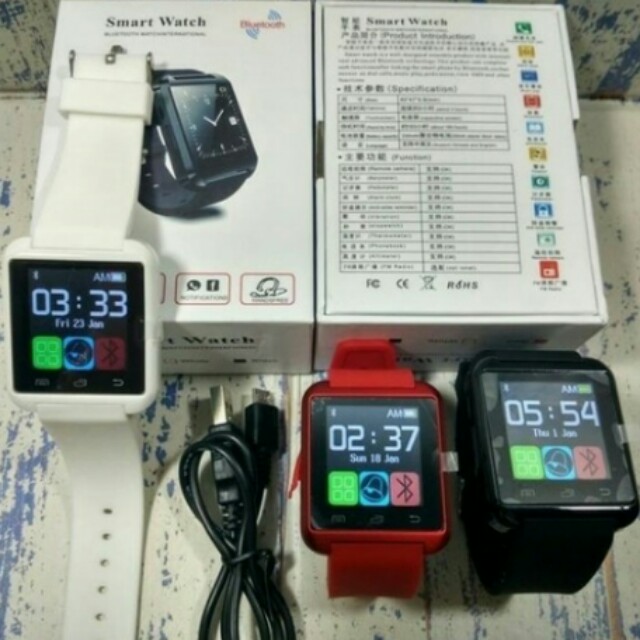This square-format color photograph features a collection of smartwatches and their packaging, artistically arranged on a table with a textured, multicolored background in hues of blue, white, and gray. Dominating the top of the image are two rectangular boxes set side-by-side. The left box shows the front with the word “smartwatch” and an angled image of a black smartwatch, while the right box displays the back with technical details and Chinese characters printed in black, along with social media icons on the margin.

At the bottom right of the frame, two smartwatches in red and black lay folded up, revealing their square faces and distinctive colored bands. Adjacent to these watches is a black power cord. On the left side of the image, another smartwatch with a white band and a square black screen is fully extended to showcase its design. 

Overall, this meticulously arranged setup emphasizes the sleek design and color variations of the smartwatches, capturing every detail with photographic realism.